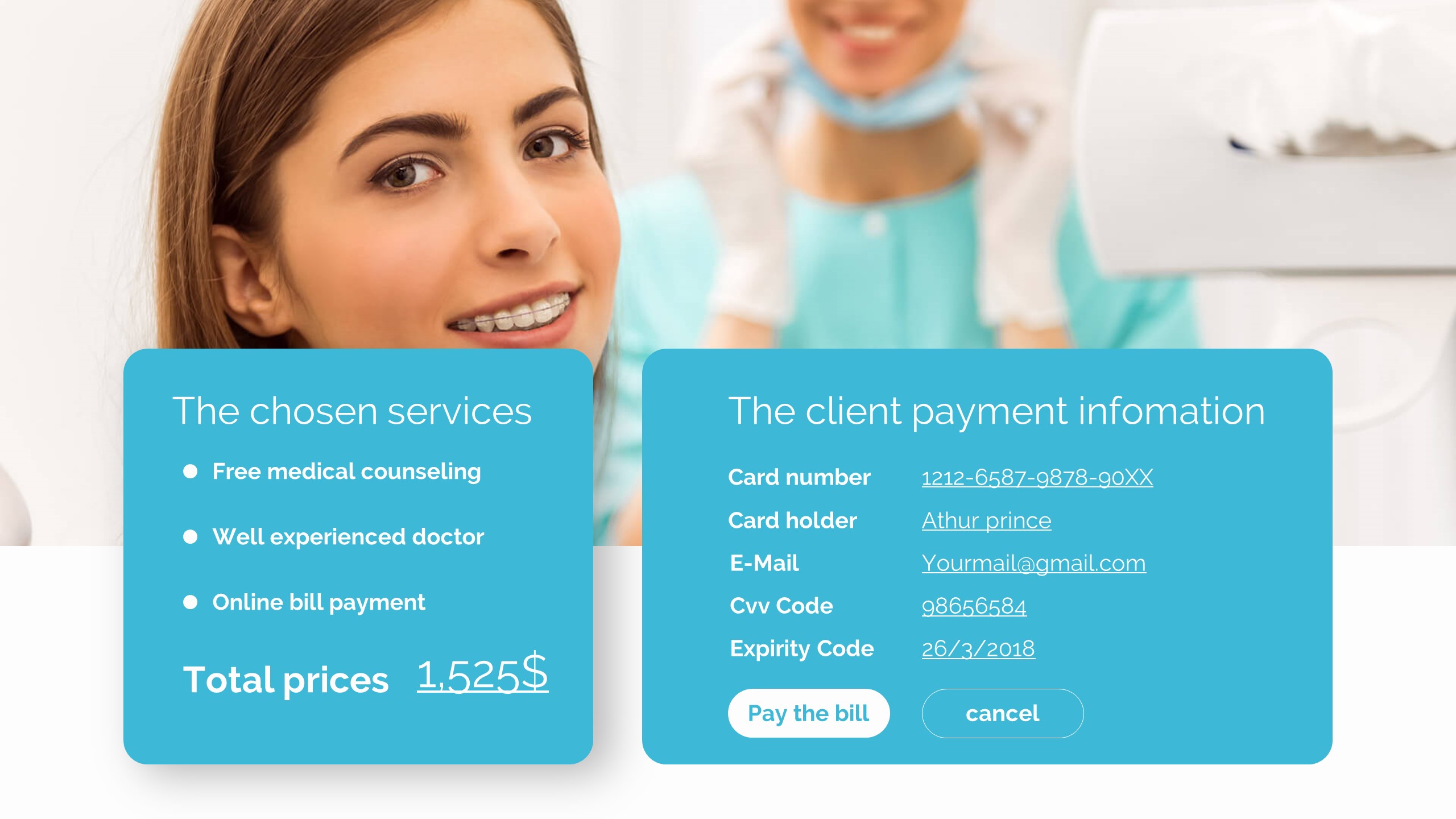This horizontally-oriented image, resembling an advertisement, prominently features two people in the background. The primary focus is on a young woman with brown hair, visible from her face down to her partially obscured chin. Her teeth are noticeably displayed, possibly fitted with a retainer. 

In the blurred background stands a medical professional, presumably a woman, who is smiling. She pulls a blue mask down beneath her chin, revealing her own smile, and is equipped with white gloves and a green top adorned with a white button.

Two blue informational boxes are superimposed on the image. The first box, on the left, lists the services provided: "Chosen Services: Free Medical Counseling, Well-Experienced Doctor, Online Bill Payment. Total Price: $1,525." The second box focuses on client payment details: "Card Number, Card Holder: Arthur Prince, Email: yourmail@gmail.com, CVC Code, Expiry Date: 26-3-2018," with options to "Pay Bill" or "Cancel."